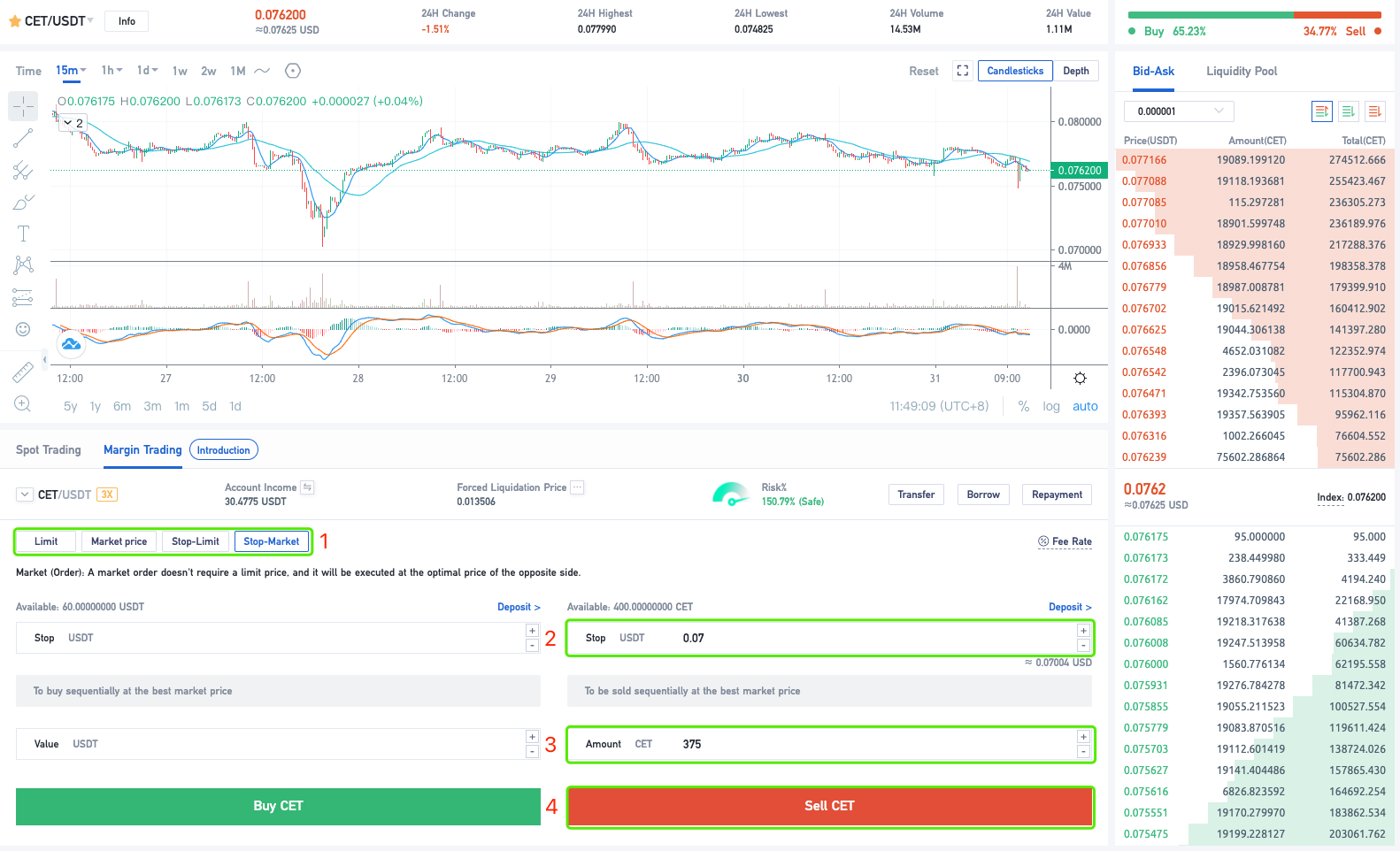This image depicts a detailed trading interface on a financial application or webpage, focusing on the trading pair CET/USDT. At the top, there is a gold star icon alongside the header "CET/USDT - Info," indicating the current trading value of CET in U.S. dollars, which is prominently displayed in orange as $0.076200. There are four or five similar items displayed across the top, but they are unreadable in this context.

In the middle section, various technical charts provide an in-depth look at the market behavior of CET, showing high, low, and moving averages. It's unclear whether these figures update hourly or daily. Midway down the page, the labels "Spot Trading" and "Margin Trading" can be seen, clarifying the trading types available.

The right column features a comprehensive list of bid and ask prices, organized in a densely packed, numerically rich format. Fields for limit and market prices are highlighted in green, with options for stop market or stop limit orders clearly marked. Options labeled one through four are highlighted, with functionalities for managing deposits, amounts, and transaction types.

At the bottom, large, easily identifiable green and red buttons labeled "Buy CET" and "Sell CET," respectively, facilitate quick trading actions. These buttons are wide and conspicuous on the left side of the interface. Overall, the interface offers a data-rich and complex snapshot of CET's price fluctuations and trading opportunities.